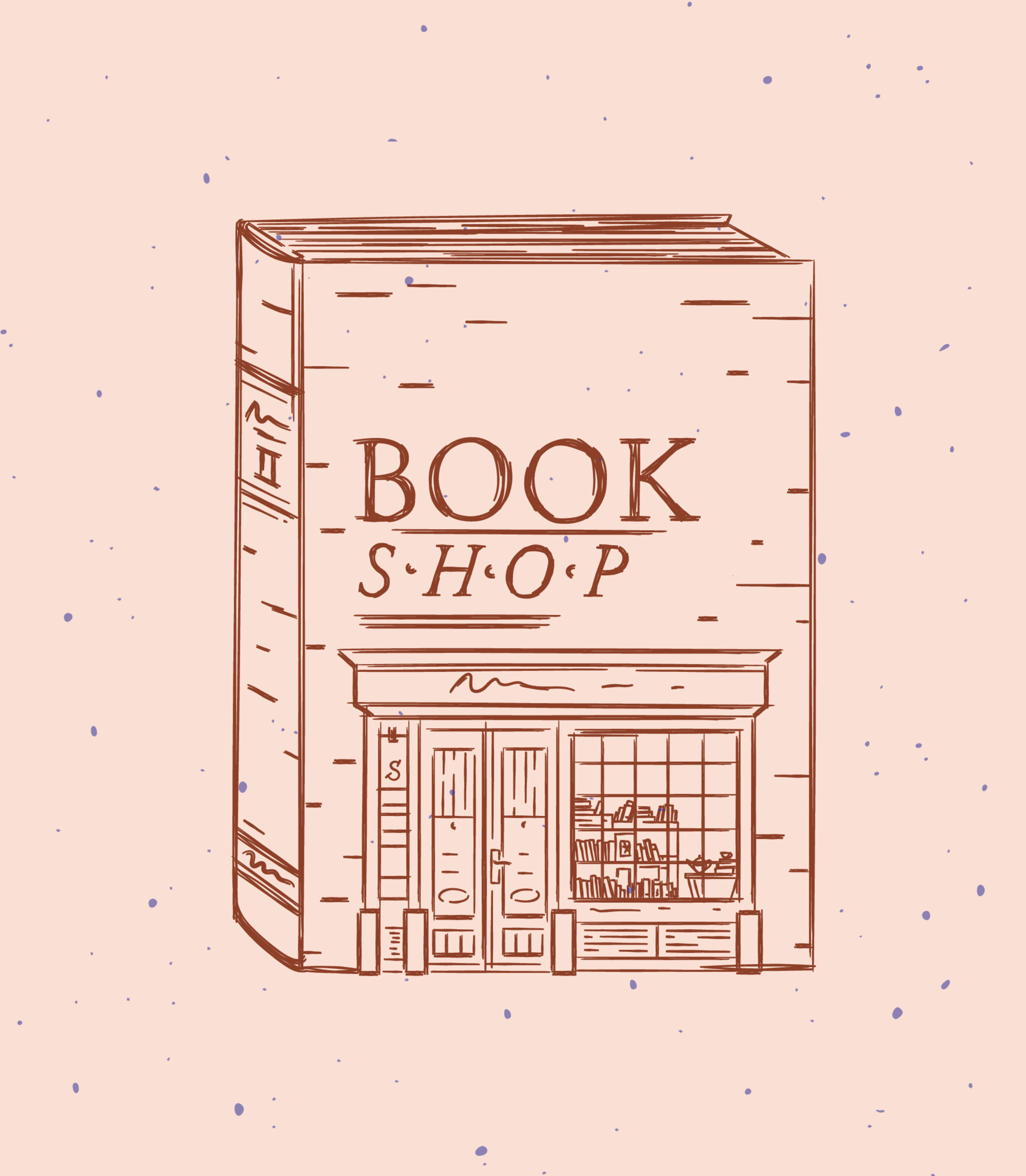The image is a tall rectangular illustration dominated by a pink background with gray speckles. Centrally featured is a whimsical, pencil-drawn depiction of a book that doubles as a bookshop's facade. The book appears to be drawn in brown or maroon ink, standing out against the colorful background. The spine of the book prominently displays the Roman numeral II, while the front cover proclaims "BOOKSHOP" in large, all-caps lettering. Below the title, there's an intricate line drawing of a bookshop, complete with double doors, an awning, and a large window. Through the window, one can see three lined shelves filled with books, adding a charming and detailed touch to this clever visual pun.